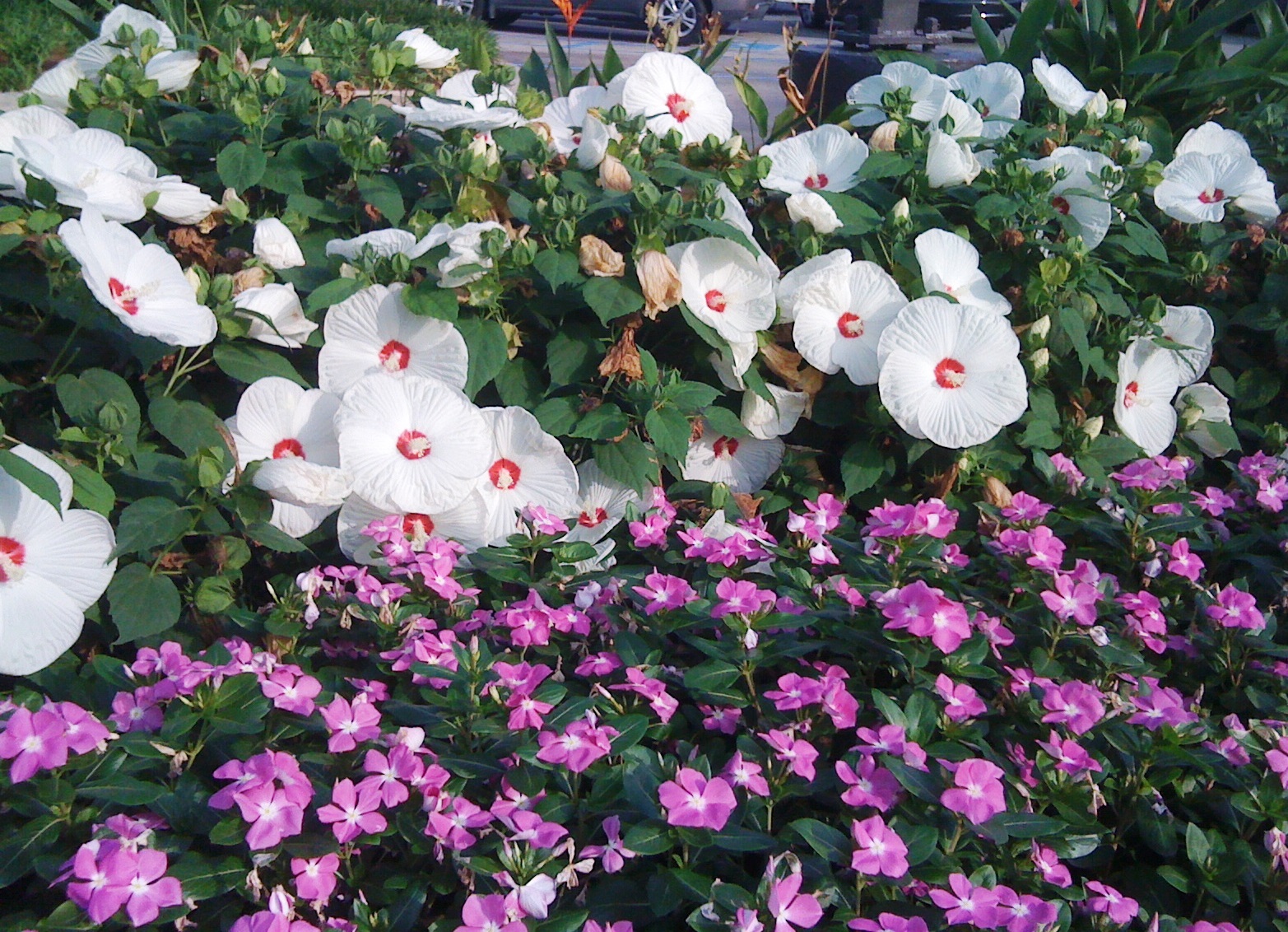The image depicts a vibrant garden scene brimming with a variety of flowers and lush foliage. In the foreground, clusters of purple flowers with delicate white centers spread across the lower portion of the scene, set against an abundant backdrop of green leaves. These flowers extend from the left to the right side of the image. Scattered above them, from the middle to the upper sections, are elegant white flowers adorned with striking red centers, some with subtle white detailing. This area appears peppered with flowers, moving from the right to the left and retreating into the background. Interspersed among these blooms are more foliage and sporadic buds, indicating ongoing growth. Towards the very top, the muted outline of a stone pathway is discernible, suggesting a garden setting, and faintly in the background, a building or house emerges, adding depth to the scene. The light in the image—whether from sunlight or perhaps sunset—illuminates the flowers, adding a natural glow to the vibrant colors and varied textures of the garden.